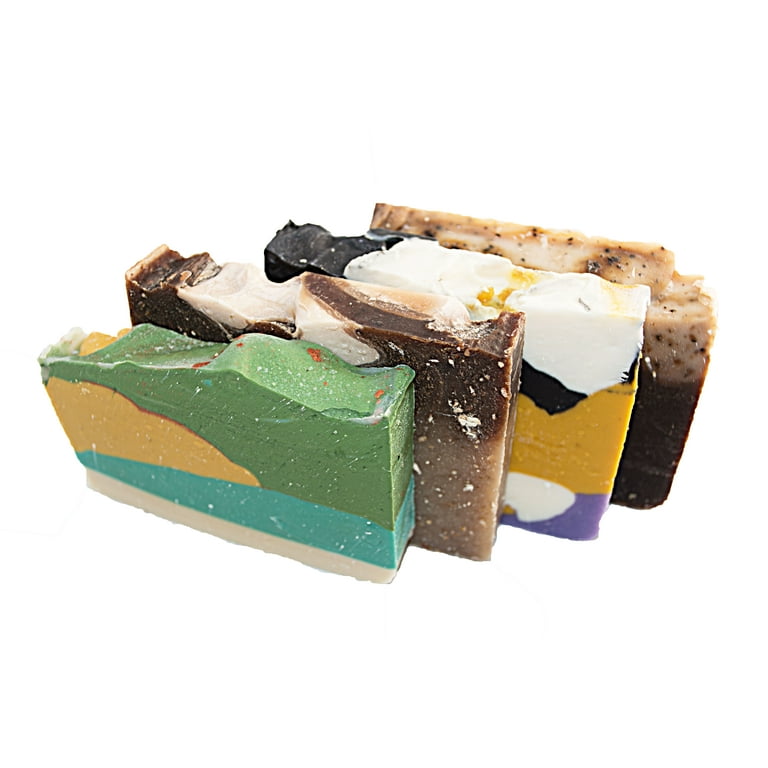The image features four handmade bars of soap, each standing on their long edge in a neat, aligned row with no spacing between them, creating a slightly offset, step-like appearance. Closest to the viewer, the first bar stands out with its distinctive color pattern: a horizontal stripe of white at the base, followed by a band of blue, a diagonal chunk of yellow from the left, and the remaining portions in green, though a section at the top is visibly broken off. The second bar, slightly behind the first, showcases a mix of browns and a touch of white, reminiscent of a chocolate bar with vanilla swirls. The third soap features a tri-color scheme with layers of white on top, yellow in the middle, and purple at the bottom. The fourth and last soap in the row presents a cream-colored top and a brown base, with notable irregularities and chunks broken off at the top. Though they may initially resemble slices of fudge due to their colors and smooth, slightly waxy texture, closer inspection reveals these are uniquely crafted, multi-colored soaps that emphasize their handmade origins. The entirety of the scene is set against a plain white background.